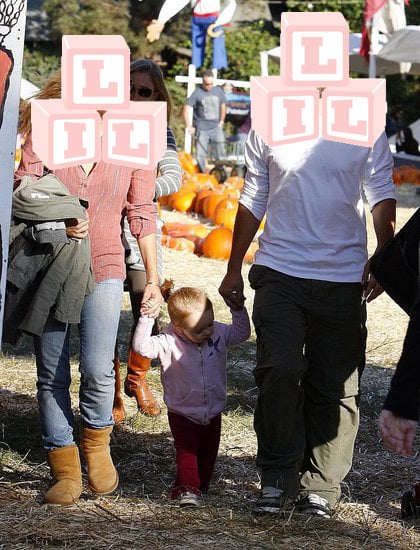In this detailed photograph of a family outing, a man and a woman are walking hand-in-hand with their young child at a pumpkin patch, set against a backdrop of scattered pumpkins and hay during the fall season. The woman, to the left, is wearing soft, velvety brown boots paired with blue jeans tucked in. She sports a long-sleeved red and white striped shirt with the top few buttons undone, holding a gray coat in one hand while firmly grasping the child's hand with the other. Her face is obscured by pink baby blocks displaying the letters L-I-L.

The child, positioned at the center, is dressed in red pants, a pink zip-up hoodie featuring a small hummingbird, and white shoes. Holding onto the child's other hand is a man on the right, clad in gray cargo pants and black shoes with white laces. Similar to the woman, his face is also covered by baby blocks spelling out L-I-L. The overall color palette of the photograph includes shades of brown, blue, red, pink, white, and the autumnal colors of the pumpkin patch. This image captures a joyous family moment amidst the vibrant and scattered elements of a seasonal outing, with a clear intention to maintain the privacy of the adults featured.